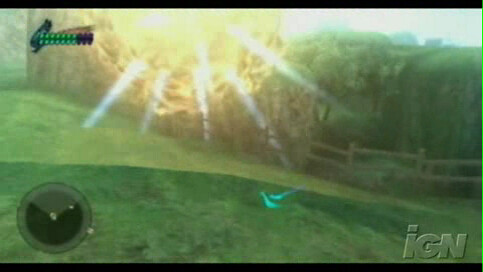Screenshot from a video game depicts a rural landscape set against the backdrop of an intense explosion. Small black borders frame the top and bottom of the image, with an "IGN" watermark positioned in the bottom right corner. In the bottom left, a circular mini-map displays a few dots and a north-pointing "N," encircled by a lighter ring. The top left hosts a partially depleted health bar, predominantly green with some black. Center stage is a vibrant country scene featuring lush green grass, a rustic brown fence, and a scattering of trees in the background. Dominating the central view is a tremendous fiery explosion, depicted with vivid yellow and white light, emanating an impressive burst of energy.